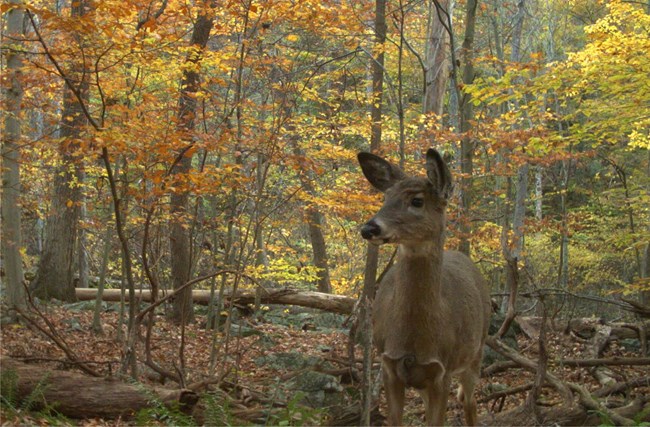The image depicts a serene woodland scene in autumn, with a central focus on a curious female deer standing slightly to the right of the center. The doe, characterized by her tall, brown ears with black tips, a black nose with a white outline, and large dark eyes, gazes to the left side of the image. She has a brown coat and stands upright, though not all of her legs are visible. Surrounding her are numerous trees adorned with vibrant fall foliage—leaves in shades of red, yellow, orange, and a few remaining green. The ground is scattered with numerous fallen leaves and branches, adding to the rich autumnal palette. A prominent log lies on the bottom left of the image, and several thin trees and twigs frame the scene, creating a natural archway around the doe. High above, the sky peeks through the dense canopy, adding a hint of blue to the otherwise warm-colored tableau. The overall atmosphere suggests a moment of alertness or curiosity, as the deer seems to be attentively listening to the sounds of the forest.